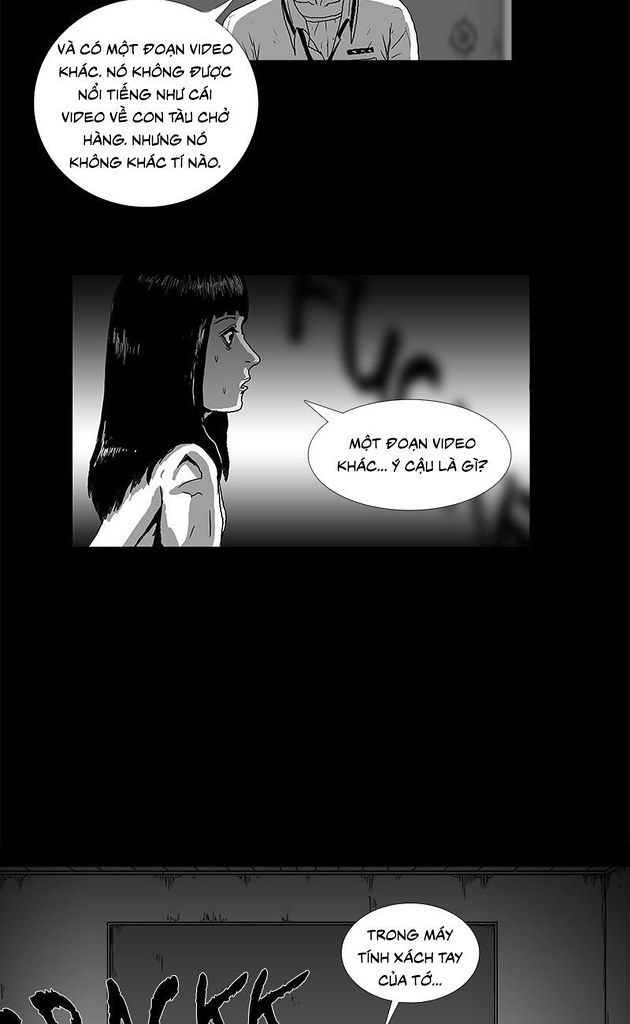The image showcases a vertical black rectangle containing three comic book panels, though only the middle one is fully visible. The text in all three speech bubbles appears to be in Vietnamese. In the top panel, partially obscured, there is a figure whose details are unclear aside from colored clothing and a lanyard. The middle panel features a young woman with shoulder-length dark hair and a white top, looking nervous as she gazes to her left. Her speech bubble appears on the right side of the panel. The bottom panel is also partially cropped out, showing a dingy wall and another speech bubble. The comic page has a predominantly dark theme, with the untranslated foreign dialogue hinting at a story rich in context.